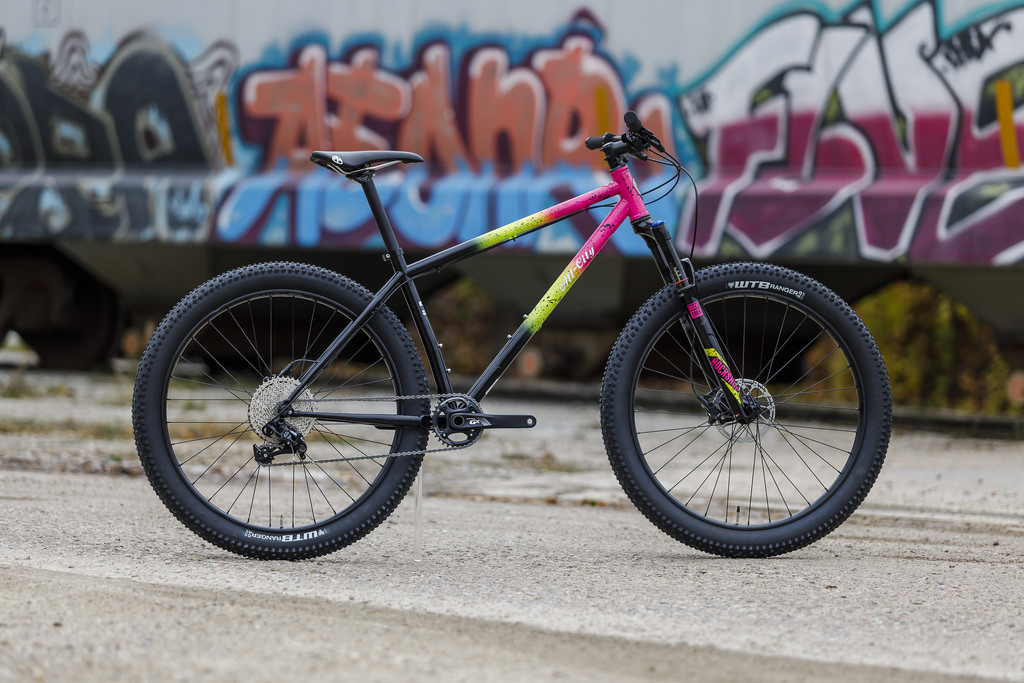The image features a colorful bicycle positioned on a concrete surface against a vibrant graffiti-covered wall. The backdrop showcases an array of graffiti, predominantly composed of bubble letters. Central to the graffiti is an unclear word rendered with the upper half of the letters in pink and the lower half in bright blue. Adjacent to this, there appears to be the word "five," with the top portions of the letters in white and the bottom in a striking magenta.

The bicycle itself sports two black wheels and has a frame with a striking gradient of colors. The lower part of the handlebars and the connecting bars start with a black hue, transitioning into a vivid yellow, and finally merging into a bright pink. The bike, potentially a mountain bike, stands out with its bold and vivid color scheme exclusively adorning the crossbars, making it a vibrant focal point against the lively graffiti backdrop.